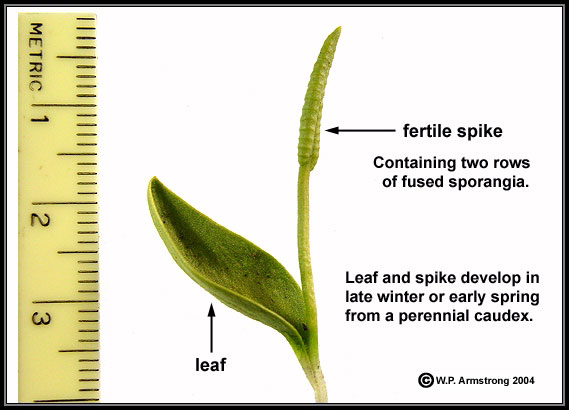The image is a detailed botanical diagram against a white background, featuring a plant with annotations and a scale for measurement. The plant's stem, colored light green, rises vertically, culminating in a conical "fertile spike" marked by small knob-like structures. This spike, resembling tiny kernels, is labeled with an arrow and text indicating "fertile spike containing two rows of fused sporangia." Beside the stem, a large, cupped leaf extends upwards and to the left, also annotated with an arrow and labeled "leaf." Below these elements, another label notes: "Leaf and spike develop in late winter or early spring from a perennial caudex." The left side of the image includes a yellow measuring tape, marked in inches and metrics, showing the plant to be approximately four inches tall. The diagram, framed in black, cites W. P. Armstrong, 2004, as the source of the information.